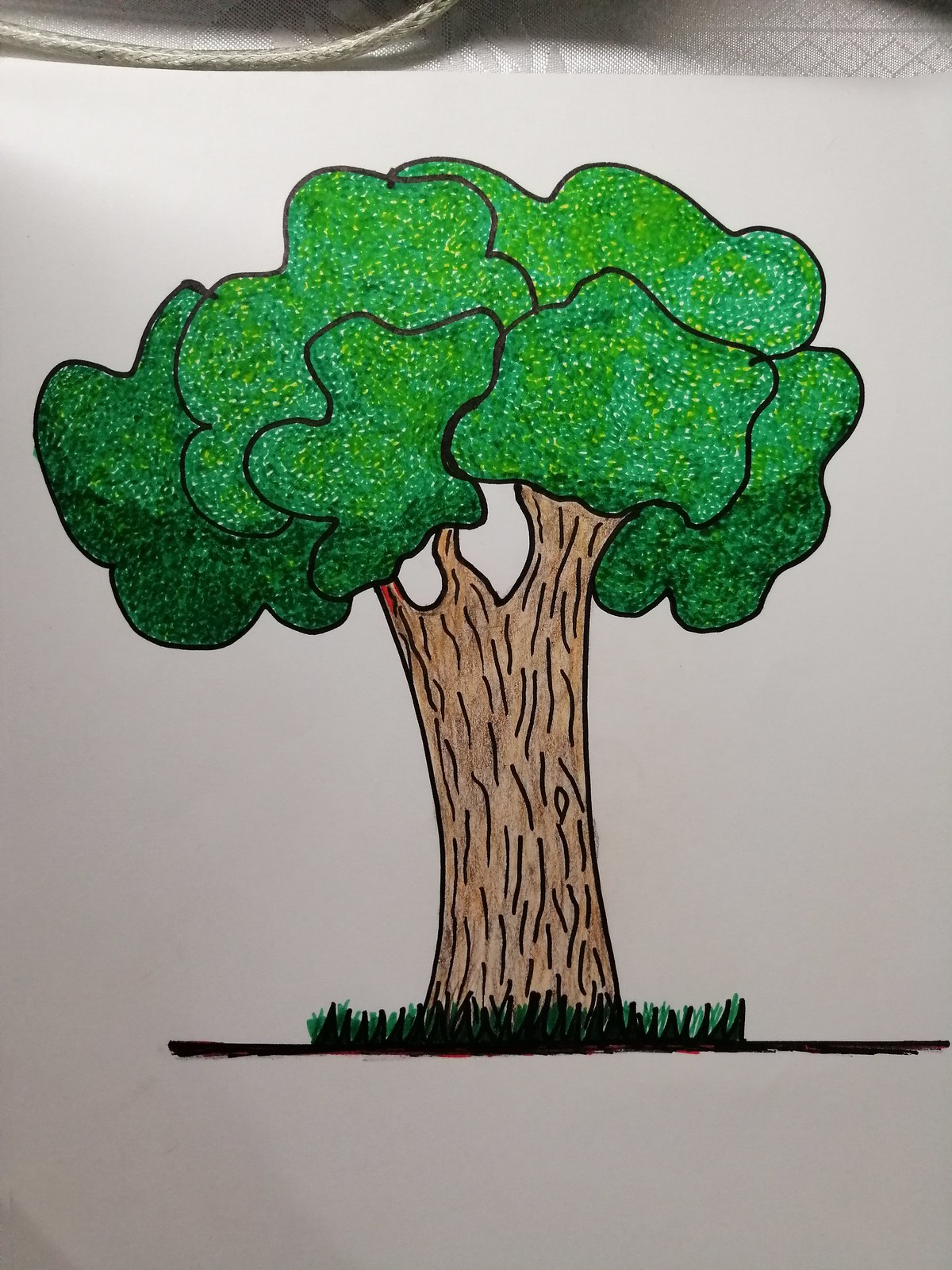This image is a colorful, stylized drawing of a tree, likely rendered with crayon or felt-tip pen, over a predominantly white background. The artwork appears to be created on paper, occupying about 90% of the frame, with the remaining 10% showing a white lacy tablecloth and a silver cord at the top left corner. Central to the image is a thick, brown tree trunk, accentuated with black lines to emblematize bark texture. The trunk bifurcates into three branches that give rise to dense, leafy clusters. These clusters are composed of vibrant green hues, interspersed with white and yellow blotches, all enclosed in blue outlines, suggestive of depth and dimension. The leaves, drawn en masse rather than individually, evoke a pointillist style, resembling bushy clouds perched atop the tree. At the base, a small patch of grass created with green and black flecks stands above a solid black line, grounding the tree within the composition.